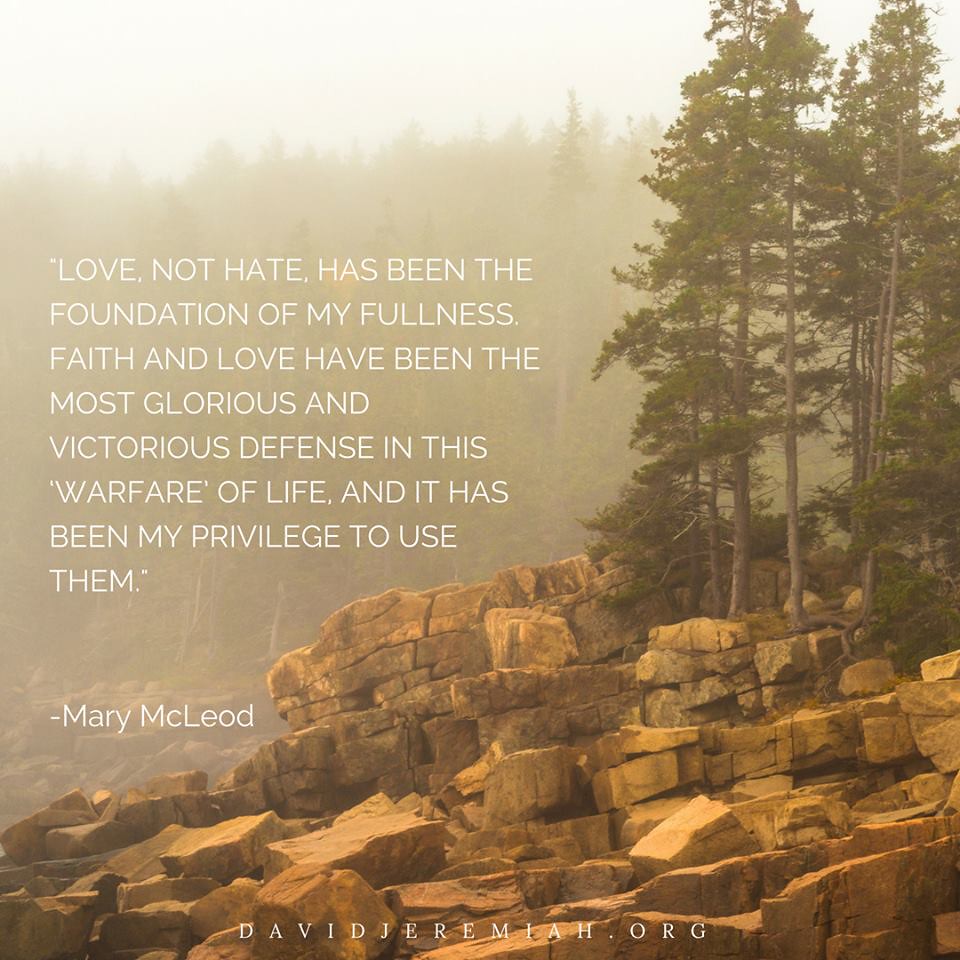This square-shaped image serves as a motivational piece that one might encounter on social media or framed on a wall. The background is a natural scene featuring flat, square-shaped rocks that climb higher to the right, resembling a rocky bluff. Interspersed among the rocks are tall pine trees, and the scene extends into a distant forest, enveloped by a foggy haze, contributing to a serene yet mystical atmosphere. Printed in white block text over the photograph is the quote: "Love not hate has been the foundation of my fullness. Faith and love have been the most glorious and victorious defense in this warfare of life and it has been my privilege to use them," attributed to Mary McLeod. At the bottom center of the image, the website DavidJeremiah.org is displayed.